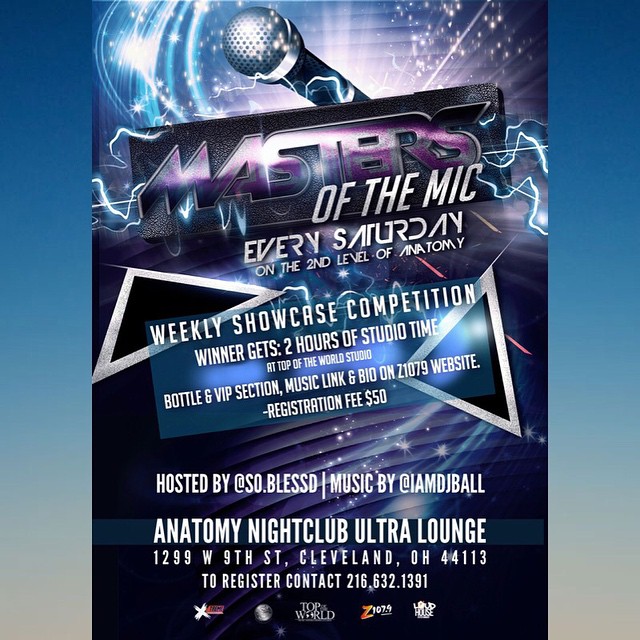The advertisement is a vertically rectangular image for "Masters of the Mic" held every Saturday at the Anatomy Nightclub Ultra Lounge, located at 1299 West 9th Street, Cleveland, Ohio 44113. The ad features vertical borders on the left and right sides that transition from a deep blue at the top to gray at the bottom. The central area of the ad includes vibrant visual elements such as blue and purple swirls of color, white streaks resembling lights, and lightning effects emerging from a large silver and blue microphone positioned diagonally from the bottom left to the top center. At the top of the ad, against a background of vertical slats, is a black rectangle with "Masters" inscribed in purple and "of the mic every Saturday on the second level of Anatomy" in gray beneath it.

Further detailing the event, a blue-bordered white banner announces a Weekly Showcase Competition where winners receive two hours of studio time at Top of the World Studio, a Bottle and VIP section, a music link and bio on the Z107.9 website. A registration fee of $50 is required. The event is hosted by @so.blessd with music by @imdjball. At the bottom of the ad, set against horizontal slats with stars and streaks of light, it prominently displays the venue name, "Anatomy Nightclub Ultra Lounge". Below that are sponsor logos: an 'X', a globe, the Top of the World logo, Z107.9, and Loud House. To register for the event, contact 216-632-1299.